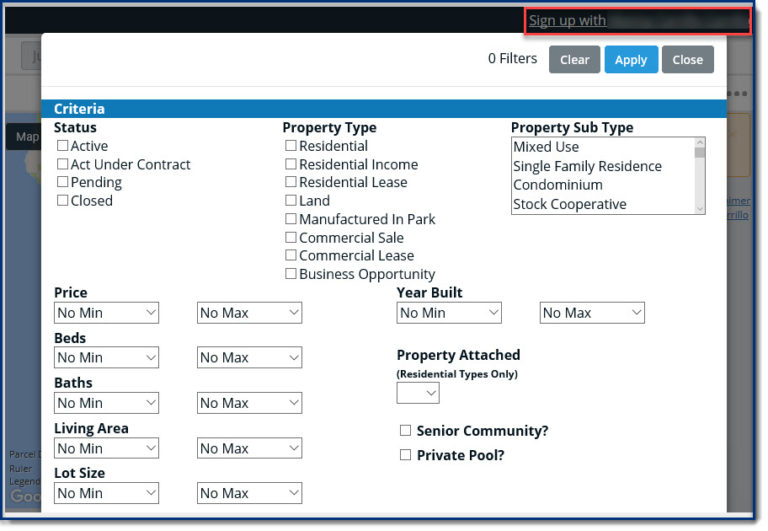The image is a screen capture of a sign-up sheet displayed as a prominent white pop-up box overlaying a shaded website background. In the background, a map is faintly visible behind the white pop-up box, which occupies the center of the screen. In the top right corner of this screen grab, there is a red highlighted box emphasizing the words "sign-up," with the next detail obscured by blurring.

The header of the white pop-up box features a broad white bar across the top. On the right side of this bar, there is text indicating "zero filters" in grey. Below this, there are three distinct blocks: a grey block with the word "clear" in white, a blue block with the word "apply" in white, and another grey block with the word "close" in white.

Directly below this bar is a blue strip running the full width of the pop-up box, featuring the word "criteria" in white on the far left. Below this blue bar, the content is divided into three columns:

**Left Column:**
- **Status:** There are checkboxes labeled "active," "act under contract," "pending," and "closed."

**Center Column:**
- **Property Type:** Checkboxes are available for "residential," "residential income," "residential lease," "land," "manufactured in park," "commercial sale," "commercial lease," and "business opportunity."

**Right Column:**
- **Property Subtype:** A scrollable list includes options such as "mixed-use," "single-family residence," "condominium," and "stock cooperative."

Further down, the image displays fields for specifying "Price" with drop-down options labeled "no minimum" and "no maximum." Additional criteria include BEDs, BATHs, living area, lot size with options to set minimums and maximums, and the year built, again with options for minimum and maximum. There are also checkboxes for specifying "property attached," "senior community," and "private pool."